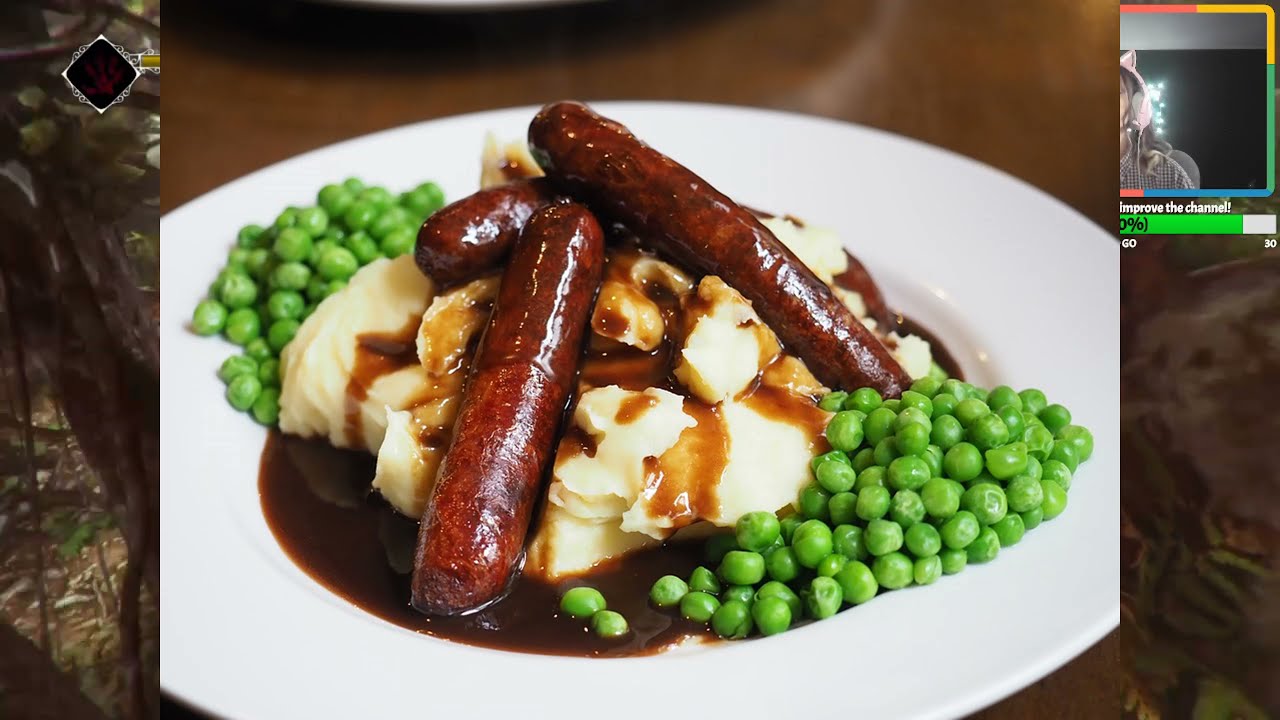This indoor photo captures a hearty meal on a large, white plate. At the center of the plate, three brown sausages sit atop a heaping mound of mashed potatoes, all generously draped with savory brown gravy. Flanking the sausages and potatoes are vibrant green peas, arranged neatly on either side. The image appears to be taken with a camera phone, as evidenced by a faint graphical overlay on the top-right corner showing a partial image of the photographer—a person wearing pink, cat-eared headphones, and a plaid brown-and-white shirt. The background features light and dark gray walls, with a brown, tarp-like material partially visible on the left side. Additionally, an overlay reminiscent of a video game HUD displays text reading "improve the channel" along with a partially visible health bar, adding a unique, modern twist to the otherwise traditional food photograph.